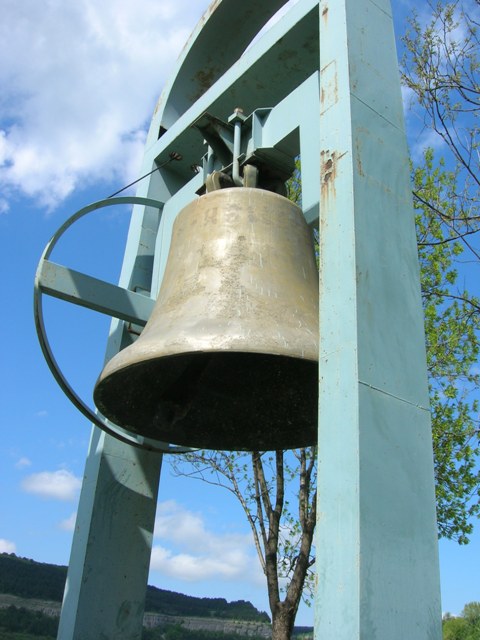This outdoor photograph captures a detailed scene with a large, prominent metal bell at its center. The bell, a substantial silver metallic structure, is suspended from a light blue, arching metal framework adorned with various industrial hardware securing it in place. In the foreground, the bell exudes a distinct presence, appearing almost copper-like in color in some descriptions. The framework, robust and supportive, is complemented by a crossbar near the top, adding to the industrial aesthetic.

Surrounding the bell and frame, a lush natural environment enhances the image's appeal. The bright blue sky fills the upper part of the background, scattered with fluffy white clouds. Tree branches adorned with fresh green leaves and buds stretch into the scene from the right and behind, contributing to the serene ambiance. Distant treetops imply a vast, possibly mountainous area extending beyond the frame. Below, a subtle stone wall or border hints at the edge of the property, grounding the scene. The overall photograph, taken during the day, blends industrial elements with natural beauty, creating a harmonious outdoor vista.